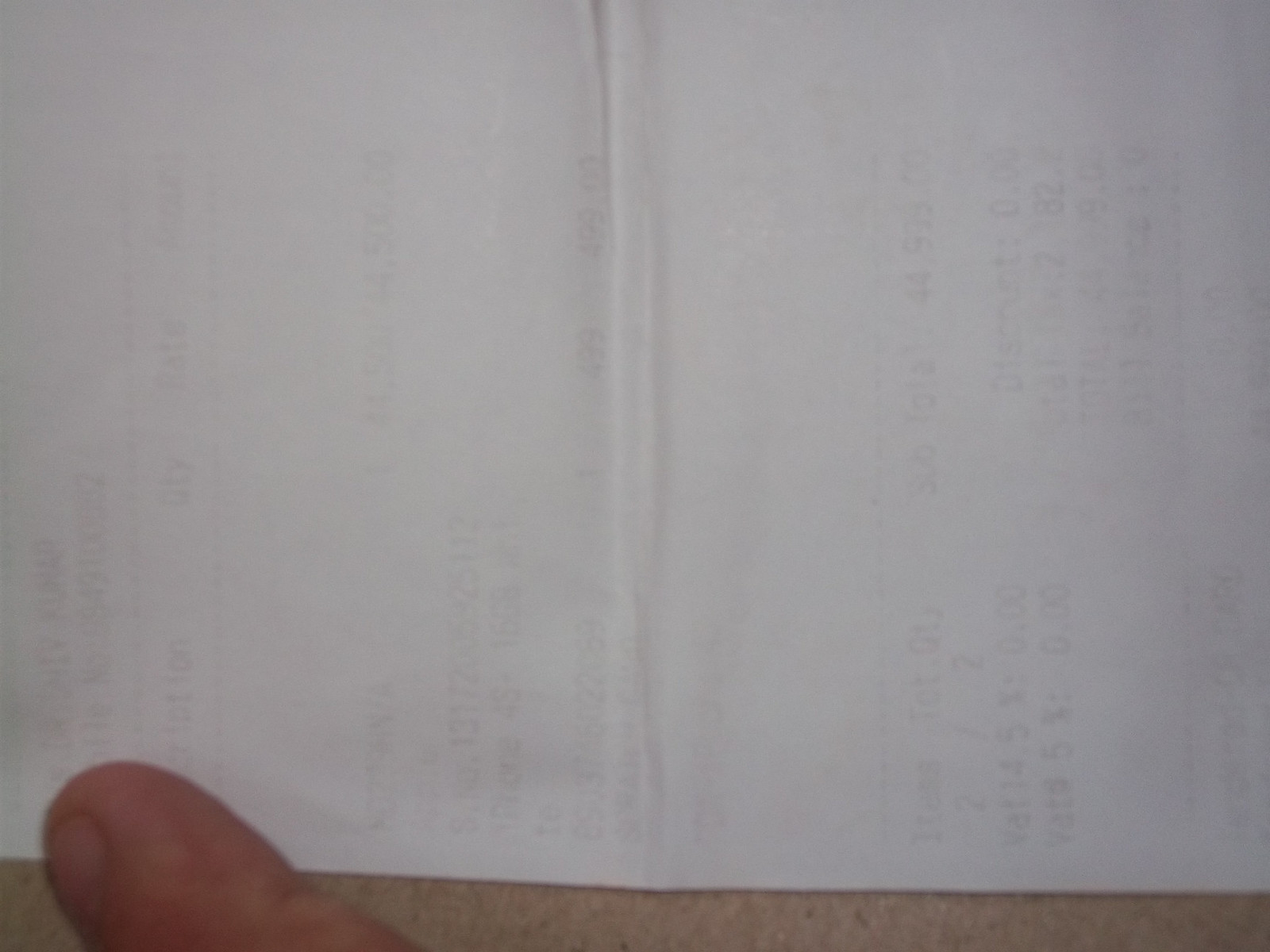The image predominantly features an upside-down receipt, which occupies most of the frame. The receipt appears slightly translucent, showing faint, faded black text indicative of shopping details such as item descriptions, quantities, rates, and a visible total amount of 44.99. The paper has a slight fold in the middle. In the bottom left corner of the image, the top third of a fair-skinned thumb, with no nail polish on the nail, is either holding or about to grab the receipt. This thumb slightly overlaps a small portion of a tannish-colored countertop, also visible at the bottom of the image.